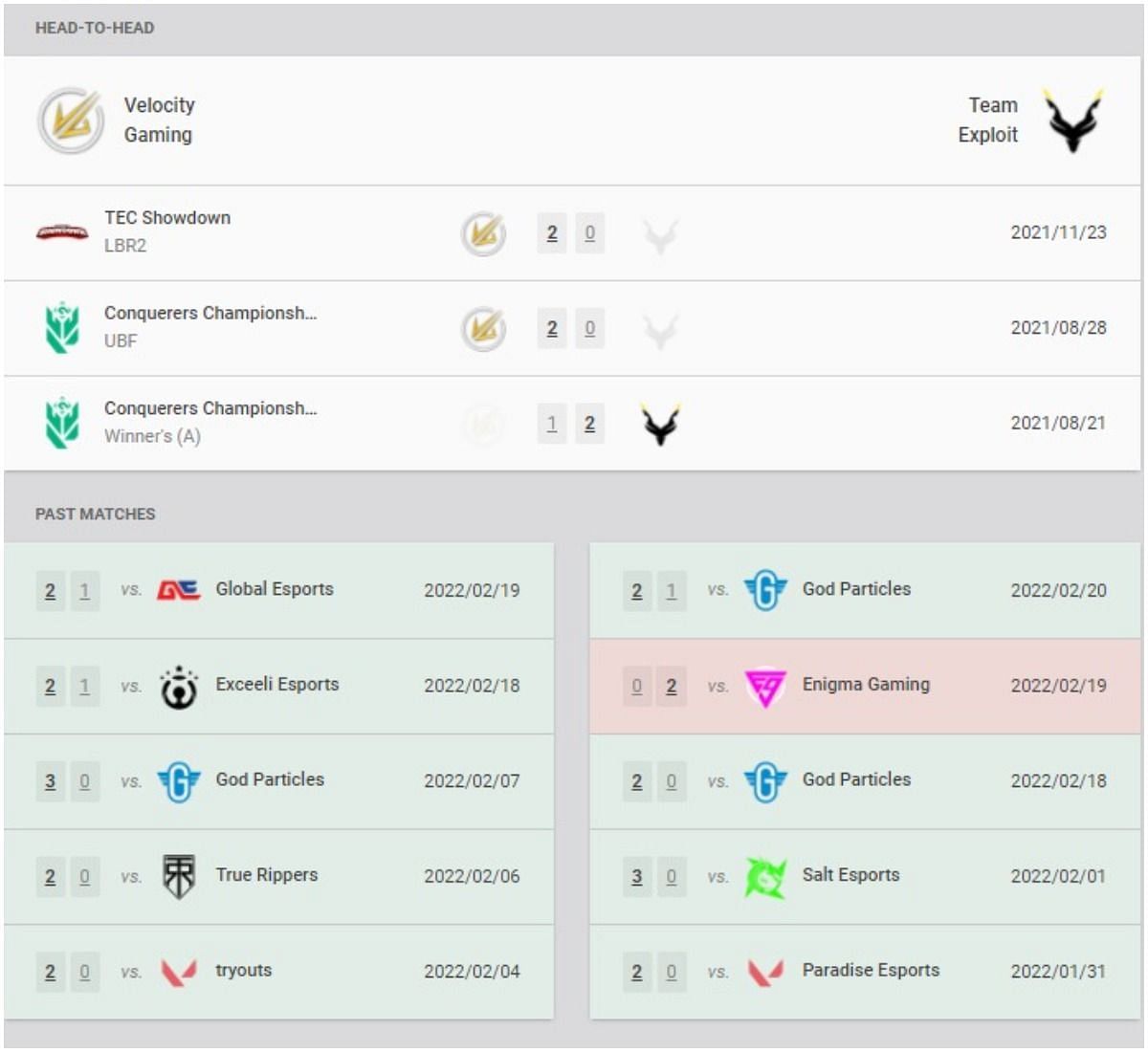The image is a detailed scorecard for a gaming match, likely for an esports tournament. On the left, there's a logo resembling a comet, representing Velocity Gaming, while on the right, there's a black symbol resembling an animal with antlers or horns, representing Team Exploit. 

At the top, "Head-to-Head" is prominently displayed, with Velocity Gaming on the left and Team Exploit on the right. Below that, "Tech Showdown LBR2" is written on a small red banner, along with the score "2-0" and the date "2021-11-23." The banner encloses the title "Conqueror's Championships," though it is truncated to "SH...". A green shield-like symbol with "UBF" is present next to this text.

Further below, the score "2-0" is prominently displayed again, with the logos for Velocity Gaming highlighted and Team Exploit grayed out. Following this is "Conqueror's Championships Winners (A)" with the same green shield logo. The numbers "1" (grayed out) and "2" (bold) are shown next to the Team Exploit symbol, along with the date "2021-08-21."

Under "Past Matches," results are listed in a downward sequence. For Velocity Gaming:
- 2-1 vs. Global Exports on 2022-02-19
- 2-1 vs. Exili Exports on 2022-02-18
- 3-0 vs. God Particles on 2022-02-07
- 2-0 vs. True Rippers on 2022-02-06
- 2-0 vs. Tryouts on 2022-02-04

For Team Exploit:
- 2-1 vs. God Particles on 2022-02-20
- 0-2 vs. Enigma Gaming on 2022-02-19
- 2-0 vs. God Particles on 2022-02-18
- 3-0 vs. Assault Esports on 2022-02-01
- 2-0 vs. Paradise Esports on 2022-01-31

This detailed scoreboard encapsulates the match history and recent performances of Velocity Gaming and Team Exploit.